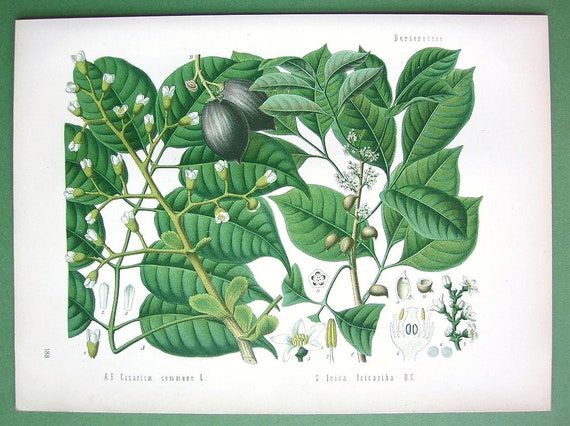This detailed poster features botanical illustrations of various plants, presented with a cartoonish style, and bordered in green. The main focus is a large plant showcasing an intricate display of green leaves, stems, and multiple stages of flower and fruit development. The central plant includes small flowers and seed-like bulbs, with some flowers still in buds and others in full bloom. Two prominent black seed-like objects dangle from the top of one of the green branches, detailed with fine, textured lines typical of seeds. Scattered around the main plant are smaller images, likely detailed diagrams presenting different stages of growth of flowers and fruits, including representations of the anemone flower. Although the text at the bottom of the poster is too small to read clearly, it appears to provide descriptions of the illustrated botanicals and their different stages.